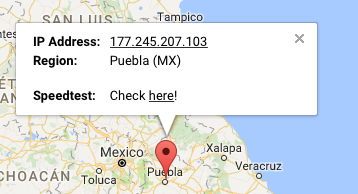A screenshot showcasing a Google Maps interface focuses on a speed test for an IP address located in Puebla, Mexico (IP: 177.245.207.103, underlined). The map is centered on a red pointer icon marking Puebla, with a white floating speech bubble extending from the pointer. The speech bubble reads: "Puebla, MX Speed Test - Check here!" with the word "here" underlined and an exclamation point emphasizing the call to action. Surrounding regions such as Veracruz, Xalapa, Tampico, and Toluca are also visible on the map. The overall image is sharp and tightly framed, displaying a portion of a water body on the right side. Notably, the screenshot lacks any branding or identifiable user interface elements, offering no clues about the company conducting the speed test.